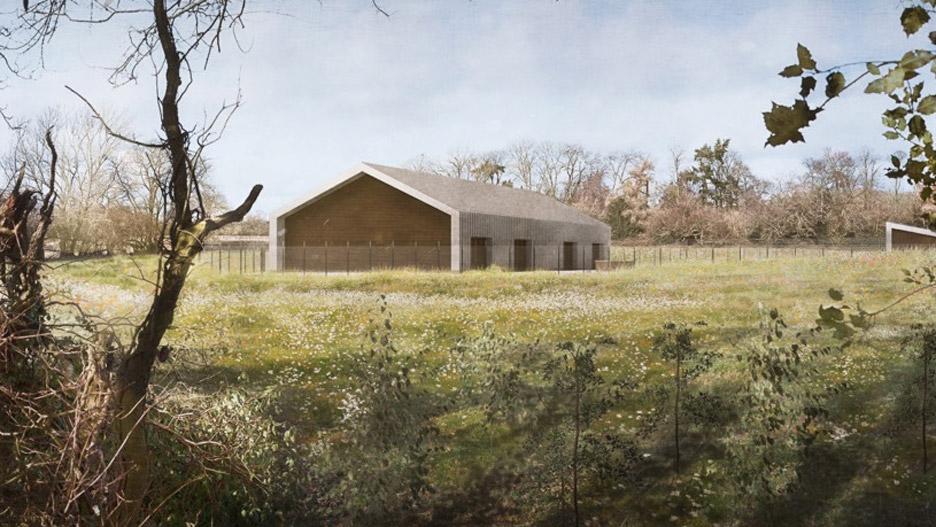This image depicts a vibrant daytime outdoor scene featuring a contemporary farmhouse at its center. The farmhouse, a large structure resembling a barn, is constructed with a combination of brown wood and concrete elements and is notable for its four large garage-like doors and a contrasting white roof. It is enclosed by a sturdy fence that surrounds the entire property. The foreground is a lush field adorned with wild grass and scattered white flowers, while the background is framed by a dense line of trees under a clear blue sky with minimal clouds. Additionally, a secondary structure with white and brown or black detailing is visible in the top right corner, adding depth to the picturesque rural setting.